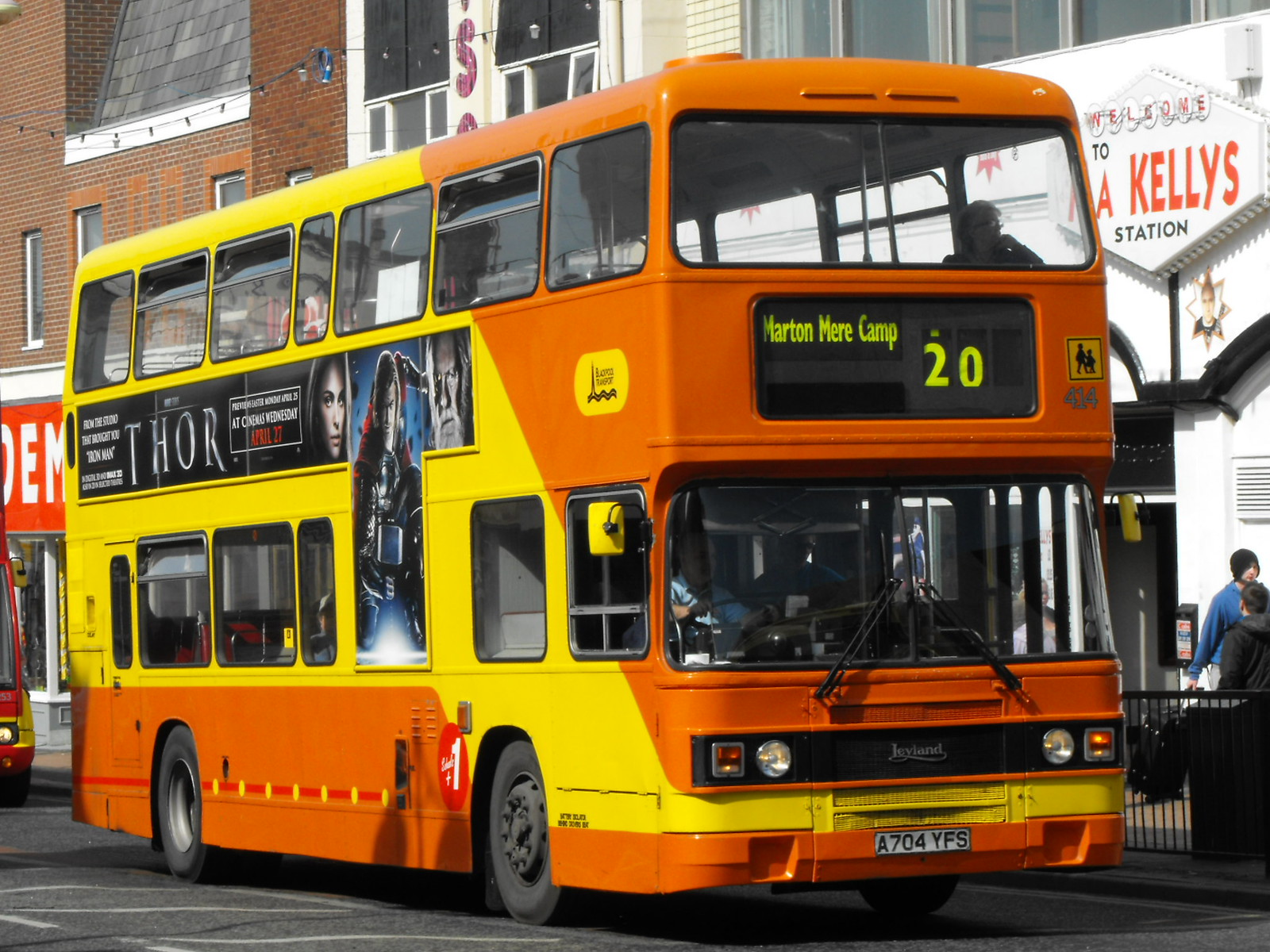In this vibrant cityscape, a striking yellow and orange double-decker bus stands out against the backdrop of tall buildings and a bustling sidewalk filled with pedestrians. The bus, prominently displaying a 'Blackpool Transport' logo, reads 'Merton Mere Camp 20' in vivid yellow on its front display screen. The license plate A704YFS is visible. Along the side of the bus, an eye-catching poster for the Marvel movie 'Thor', advertises its April 27th release. Inside the bus, the driver is visible through the window, while a passenger can be seen on the top deck near the front. The backdrop features a mix of architectural styles, including a white building labeled 'Kelly Station' and several other brick structures, adding to the urban charm of the scene.